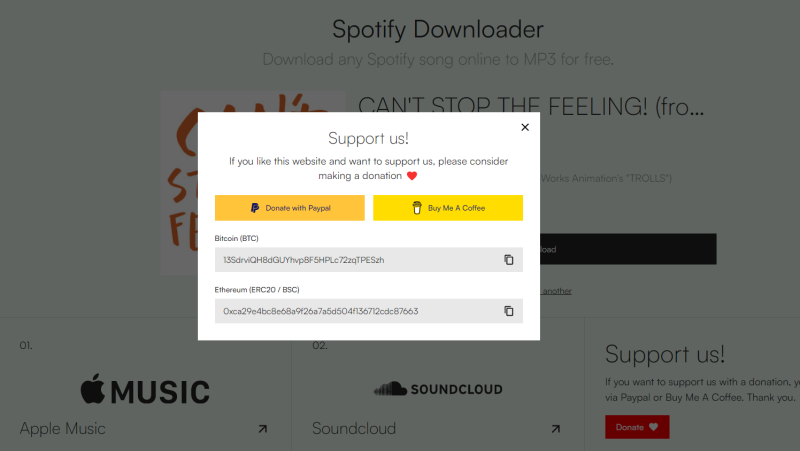This is an image of a website with a gray background, likely altered due to a prominent pop-up window at the center. The webpage header reads "Spotify Downloader," followed by a subtitle: "Download any Spotify song online to MP3 for free." The logo, partially obscured by the pop-up, is in red. Beneath the header, the text "Can't Stop the Feeling" appears, but another phrase next to it is incomplete due to the pop-up intrusion. A clickable search bar is partially covered by the pop-up as well. 

In the bottom left corner, icons with labels "Apple Music" and "SoundCloud" are visible, each linked to their respective services. To the right, there's a section inviting donations, with options for PayPal and "Buy Me a Coffee," along with a "Donate" button. Above the donation section, a similar message is displayed with options for Bitcoin and Ethereum contributions, followed by a heart symbol.